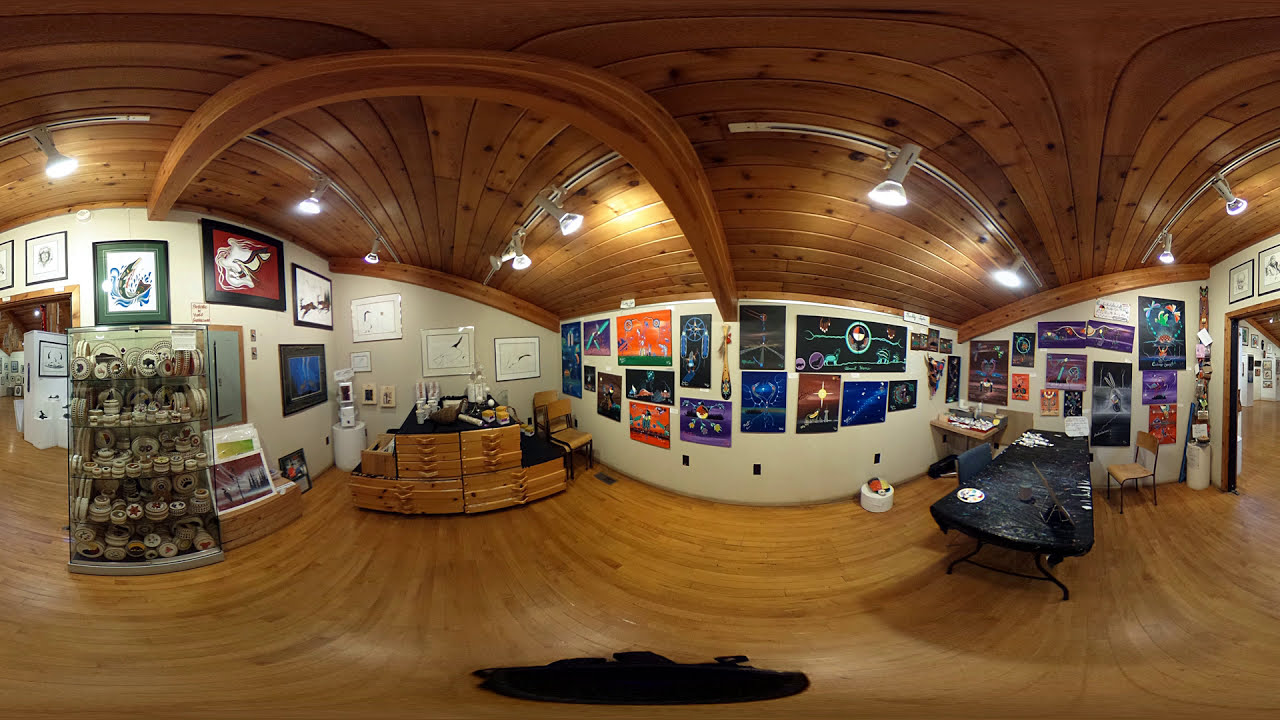This photograph, potentially captured by a surveillance or a 360-degree camera, offers an eclectic view of what appears to be a gift shop, art gallery, or art store. The space features a brown paneled wooden ceiling and floor, both with arched, curving patterns that create a surreal, almost drugged-out visual effect. The walls, painted white, curve downward, following the ceiling's dynamic arches. They are adorned with a diverse array of framed and unframed artworks in various colors such as orange, black, blue, purple, and brown. Display shelves throughout the room house an assortment of products, possibly clay objects, all uniformly organized. Overhead lighting punctuates the room with bright white spots, adding to the glassy, distorted ambiance. A table and chair are positioned within the space, hinting at its functionality beyond mere display.